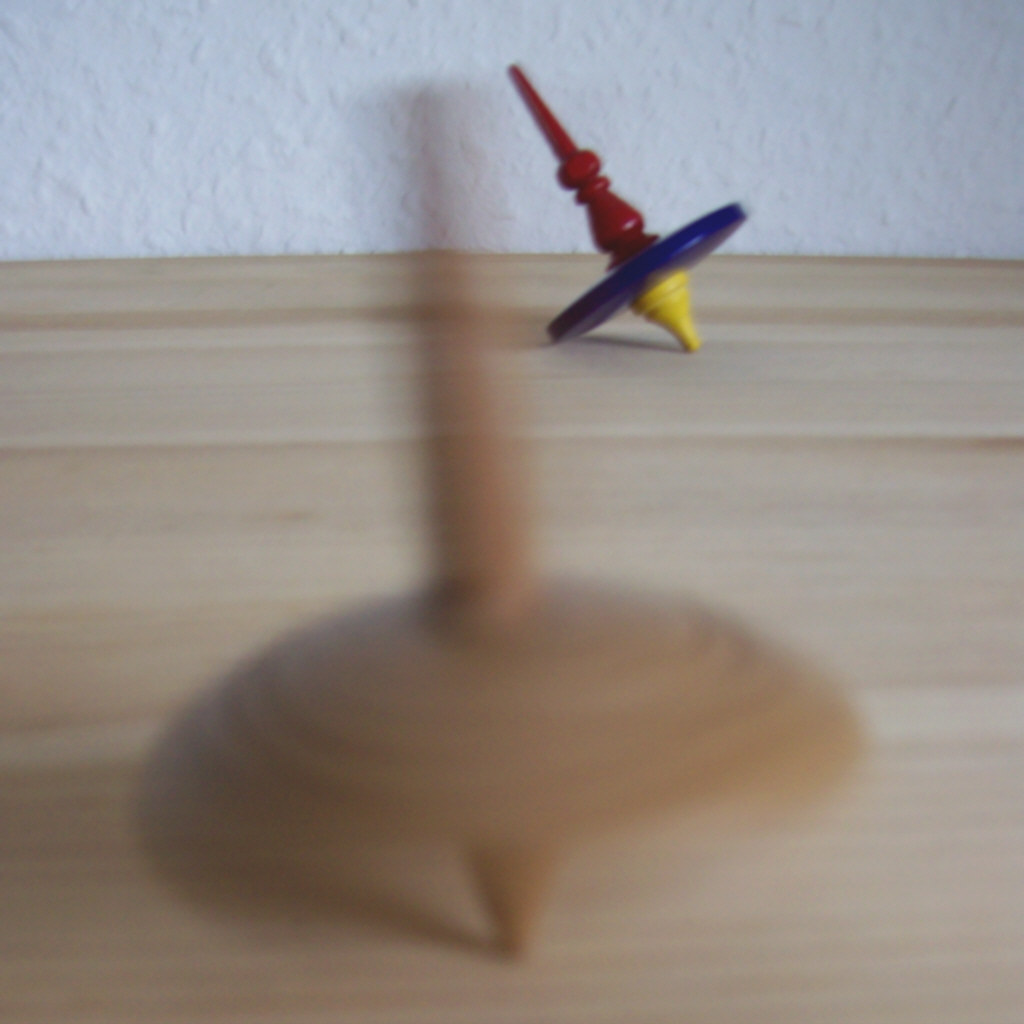This photograph captures two spinning tops poised on a smooth, almost white wooden surface. The top in the forefront, made of plain wood, is caught in mid-spin, appearing very blurry which indicates its rapid motion. This top has a light wood finish, slightly darker than the surface it rests upon, and features a typical design with a narrow bottom piece, a rounded middle, and a stick on top for spinning. In the background, approximately a foot away, another top catches the eye with its vibrant colors: a yellow spinning part, a blue deck, and a red handle. This second top is in the process of tipping over, indicative of its spin coming to an end. Behind the spinning tops is a white concrete wall with a textured, bubbly stucco design, adding a subtle backdrop to the scene. The overall composition highlights the dynamic motion and colorful contrast between the two toys.